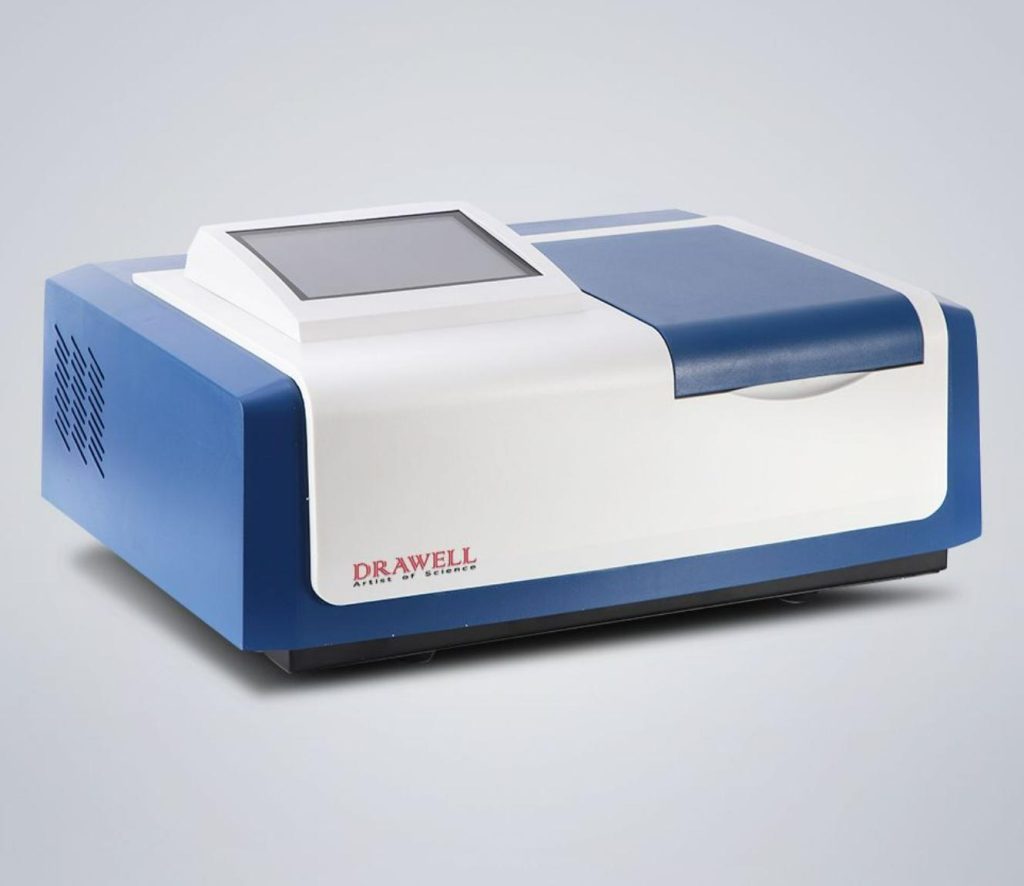The image depicts an old rectangular electronic device with a blue and white color scheme, positioned on a slightly off-white surface. The device is angled slightly towards the right. The back left side of the machine features three columns of slanted lines, likely serving as exhaust ports. On top, the device has a small display screen slanted towards the viewer, which is currently blank. The top surface is divided into two sections, blue on the right and white on the left with the display screen. On the right side, there is a vertical blue rectangle hatch with a groove underneath, possibly for opening. At the bottom left of the front, the text reads "DRAWL, Artist of Science" in red.